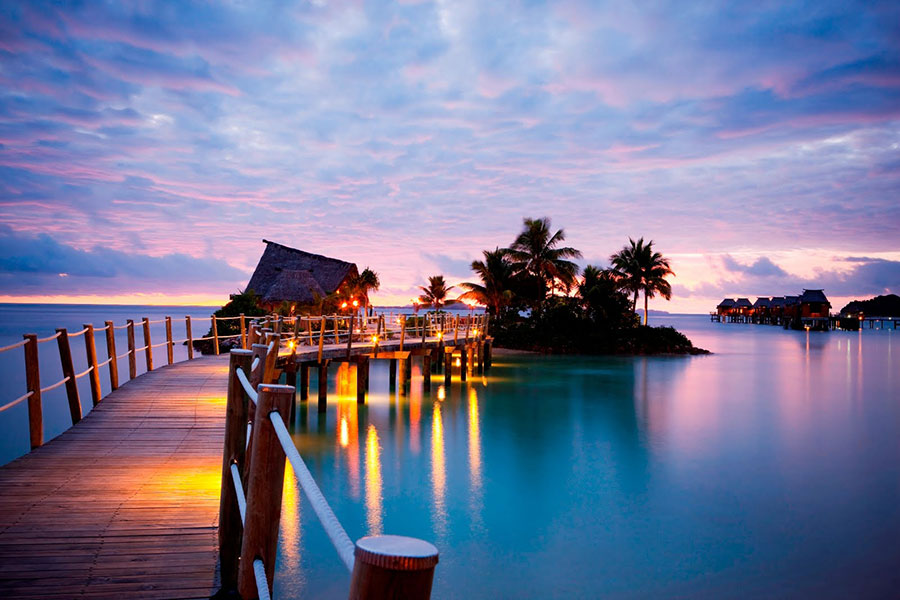In this photograph taken at sunset in a tropical beach resort, a tranquil cove with crystal-clear, calm seawater stretches out under a sky filled with hues of pink, purple, and blue due to the sun dipping below the horizon. At the center, there is a small island adorned with the dark silhouettes of palm trees and some houses or bungalows. A rickety yet charming elevated wooden bridge, lined with lights that cast shimmering reflections onto the blue and pink-tinged water, leads from the foreground to the island. The bridge, with its wooden poles and white rope handrails, guides visitors to bungalows built on stilts, standing about six feet above the serene ocean. On the right side of the image, another row of similar stilt houses floats charmingly above the water, enhancing the idyllic scene.